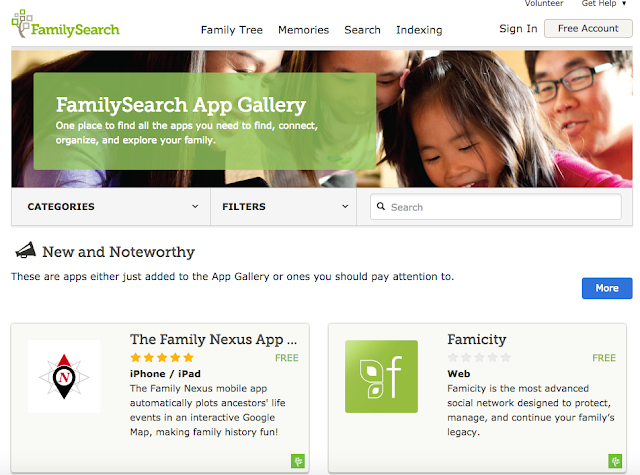This image, sourced from a webpage, prominently features a family tree graphic with geometric shapes at the top, alongside the "FamilySearch" logo. Below the logo, the menu options "Family Tree," "Memories," "Search," and "Indexing," are clearly displayed. In the upper right-hand corner, there's an area for users to sign in or create a free account, and labels for "Volunteer" and "Get Help." 

The main section of the image shows a cheerful family of four, potentially two young girls, a woman, and a man, all smiling warmly. Their expressions suggest happiness, but the context of their activity isn't visible. Overlaying this family picture is a semi-transparent green rectangular box that reads "FamilySearch App Gallery." It describes the gallery as a central hub for finding, connecting, organizing, and exploring family-related apps, with sections for categories, filters, and search functionalities.

Additionally, the box highlights a "New and Noteworthy" area for showcasing recently added or important apps, with a clickable "more" button for further exploration. At the bottom of the image, there are two blog-like sections providing additional resources or articles for users to click on.